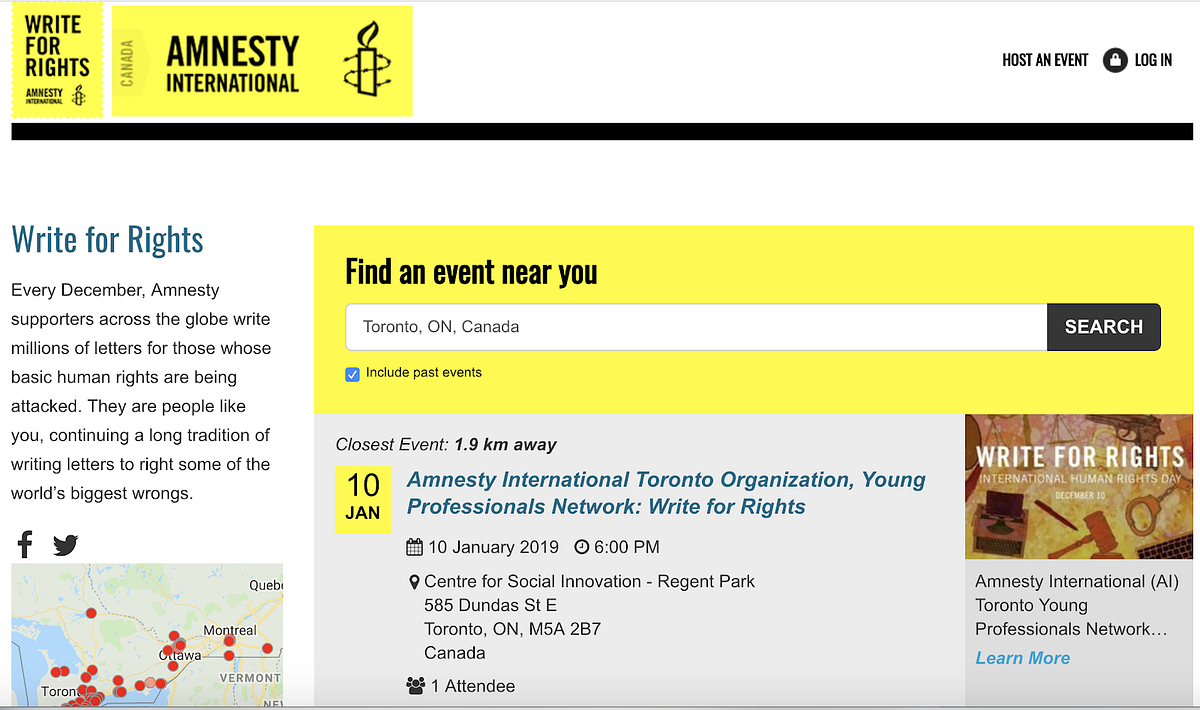Here's a detailed, cleaned-up caption for the image:

---

The image, sourced from a website, features a white background. At the top left, a thin horizontal gray bar stretches across the screen. Adjacent to this bar on the left, there's a yellow rectangle. Within the yellow rectangle, the words "RIGHT" appear in bold black text, stacked above the words "FOR RIGHTS." Below this, in smaller print, "Amnesty International" is written, accompanied by the organization's logo— an emblem of a candle circled by barbed wire.

Running vertically along the left side is another yellow strip that reads "CANADA" in bold, capitalized black letters. To its right is the same Amnesty International logo. Beside this, in smaller but bold black letters, it says "HOST AND ADMIN." A black square with a white lock icon symbolizes the login option, marked by the word "LOGIN" to the right.

Beneath these elements, a thicker black border spans the width. About an inch below, "RIGHT FOR RIGHTS" is clearly written in blue, spelled out as "R-I-T-E-F-O-R-R-I-G-H-T-S." Following this, eight lines of text detail the organization’s mission concerning human rights.

To the immediate right of this section, social media icons for Facebook and Twitter appear in black, alongside a small map dotted with red pins. Next to "Right for Rights," another yellow rectangle signals users to "FIND AN EVENT NEAR YOU" in bold, black text. Below this, a horizontal search bar runs across the screen, transitioning from white to black on the right end, where it says "SEARCH" in white text.

At the image's bottom, a blue border extends downward, providing additional information about the nearest event, including its location and date.